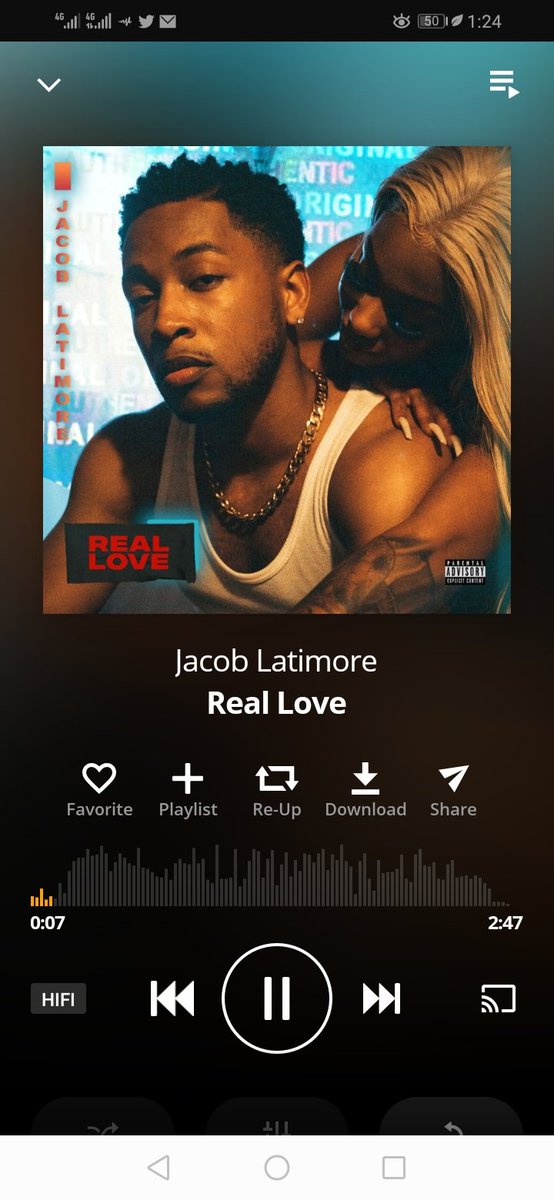The image is a detailed screenshot from a person's cell phone, focusing on a music player interface. At the top of the screenshot, there is a black status bar displaying various icons: coverage signal, Twitter, email, a battery icon showing 50% charge, and a time indicator reading 1:24. The background of the screenshot is predominantly black, providing a striking contrast to the vibrant album art featured in the center.

The album art showcases a young African-American man gazing directly at the camera, exuding a confident presence. He is dressed in a white tank top and complemented by a gold chain around his neck. Behind him, a woman with long, wavy blonde hair and long fingernails leans down, peering over his left shoulder. The composition of the album cover is enhanced by the text "Jacob Latimore" written vertically along the left side in bold letters.

On the bottom left corner of the album art, a black box with red text spells out the title of the song, "Real Love." Opposite this, on the bottom right corner, is the recognizable "Parental Advisory" sticker. Beneath the album art, the interface continues to provide details about the song such as the artist's name, "Jacob Latimore," the song title, "Real Love,” and various user options: favorite, playlist, re-up, download, and share.

The progress bar indicates that the song is currently at the 7-second mark out of a total duration of 2 minutes and 47 seconds. At the very bottom of the screen, there are classic media control buttons including 'back', 'pause', 'forward', and a 'full-screen' option. The overall orientation of the screenshot is portrait, being taller than it is wide.